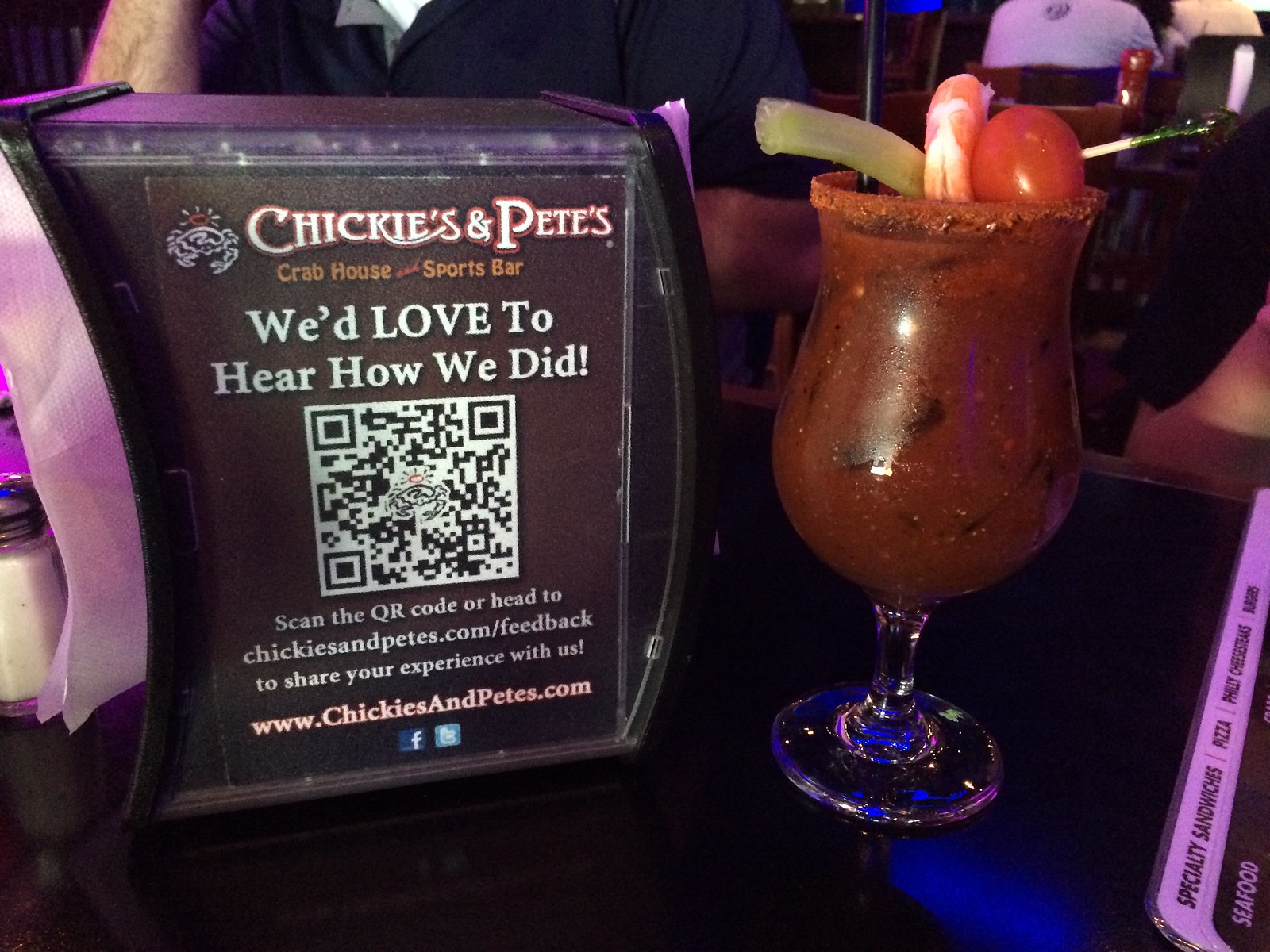This color photograph, taken in landscape orientation, captures a detailed scene at a restaurant, specifically at a table in Chickies and Pete's Crab House and Sports Bar. The focal point is an upright napkin holder on the tabletop, which features an advertisement on its side. The advertisement reads: "Chickies and Petes, Crab House and Sports Bar. We'd love to hear how we did," followed by a QR code for scanning and instructions: "Scan the QR code or head to chickiesandpeets.com/feedback to share your experience with us!" Additionally, there are a Facebook and Twitter logo, with the complete URL "www.chickiesandpeets.com" displayed in pink beneath. 

To the holder's immediate left stands a salt shaker, and a single napkin pokes out from the holder's top. On the right side of the napkin holder is a red cocktail beverage, likely a Bloody Mary, garnished with a stalk of celery, a shrimp, and a cherry tomato. The glass is adorned with a black straw and has a rim that appears to be seasoned. A partial view of the menu is visible next to the drink, cut off at the edge of the photograph.

In the background, a man is seated at the table, and other patrons are visible, though cropped out partially at the top. The ambiance captures the realism of a lively restaurant setting, illustrating the establishment’s attention to customer feedback and engagement through the promotional graphics on the napkin holder.